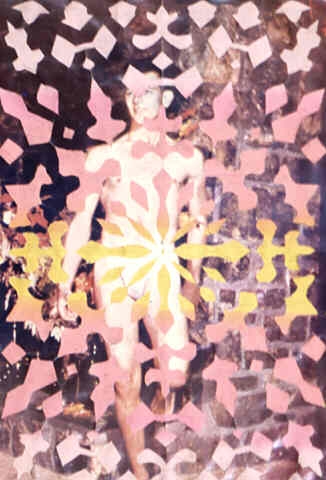The image features a manipulated black-and-white photograph of a smiling, dark-haired man with a lean build, seemingly nude except for a cloth covering his genitals. He stands against a backdrop where a stone or brick wall is partially visible. The man’s complexion is predominantly white, but his legs from the knees down exhibit a natural skin tone. Overlaid on this photograph are various geometric shapes, primarily irregular rhombuses, that resemble interconnected pieces or elements akin to the tops of temple structures and lava lamp patterns. These shapes are densely peppered throughout the image, transitioning in color from an orange-yellow center to pink, and finally to a lighter pink or white towards the edges. The overall effect creates a contrast between the vivid, almost surreal patterns and the simplicity of the monochrome photograph beneath.